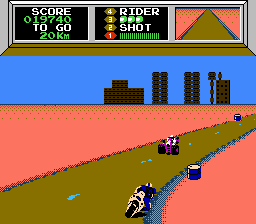The image appears to depict a video game screen showing a racing scenario. At the top of the screen, there is a scoreboard displayed against a black background. The scoreboard shows the following details: "Score: 019740" and "Distance: 20 km".

To the right of the score, also on a black background, there are indicators labeled "Rider" with three green dots next to it, and "Shot" which is followed by the number "1" in red, complemented by green lines.

The rest of the screen features a vividly colored racetrack. The ground is colored in hot pink, creating a stark contrast against the racing lanes. The two-lane road itself is an olive green color, with turquoise dashed lines serving as lane dividers.

The racers on the track are distinguishable by their attire and vehicles: one competitor is on a white motorcycle, donning a black suit and a white helmet. The other racer, who is more difficult to discern, appears to be wearing a white suit. However, the type of vehicle this second competitor is riding remains unclear.